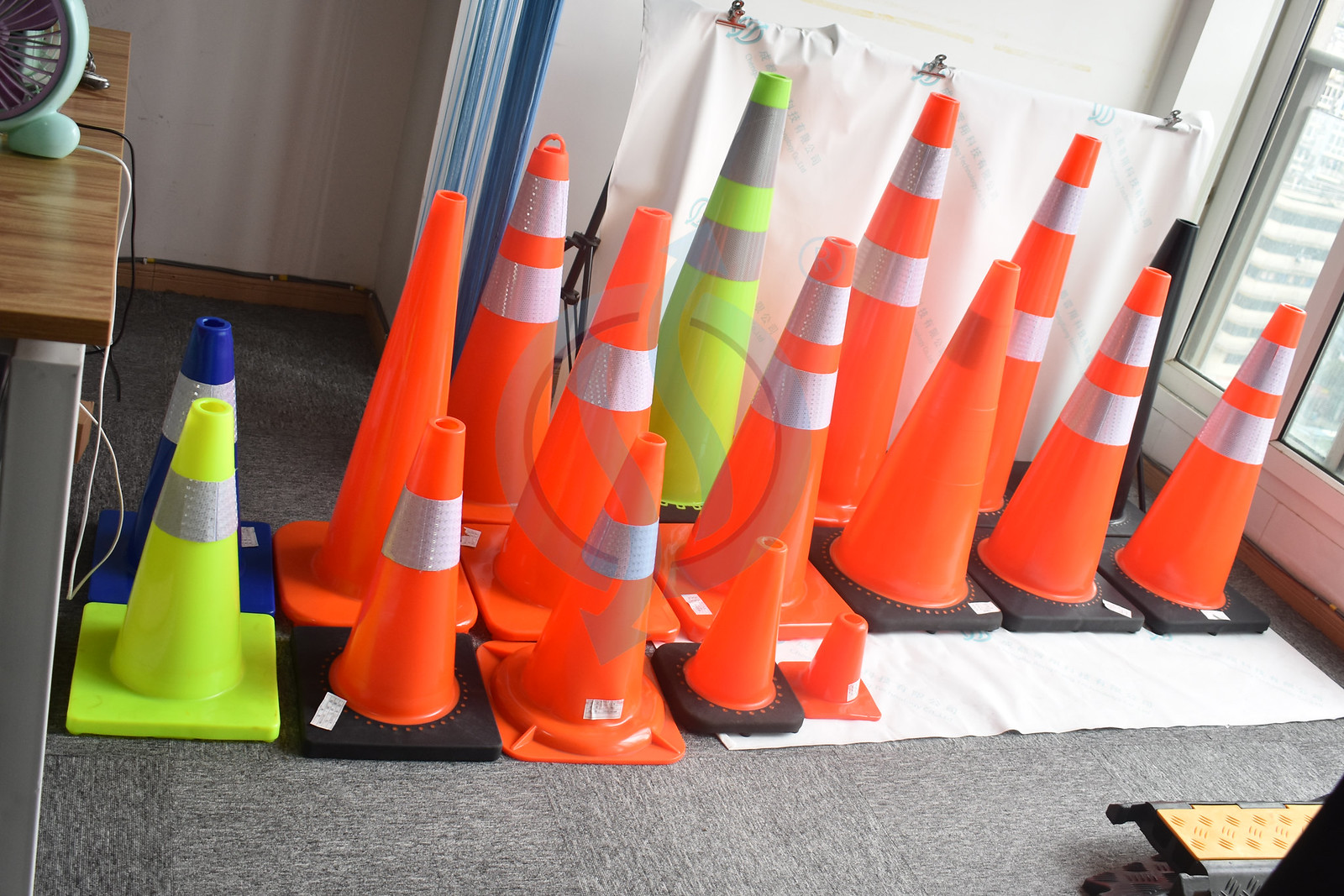The image showcases an interior room with gray carpet flooring, arranged in three neat rows of parking cones, predominantly orange. Among these cones, various sizes and designs are evident. To the left, small neon yellow and dark blue cones with silver tips stand out, while a large orange cone with a smaller one in front adds to the array. Another notable cone is a large orange one with two silver stripes on its top. The middle row features a large orange cone with a silver stripe near the top and a small cone in front of it, also with a similar stripe. In the back row, a neon yellow cone with two neon gray stripes is positioned in front of an orange cone with two silver stripes, accompanied by other small orange cones with either black or orange bases. The rightmost row includes another large orange cone with two gray stripes and a black base, alongside shorter cones with similar striping and bases. Amidst these primarily orange cones, two bright green cones with white stripes, and a blue cone with a white stripe, add diversity. The room's background includes a portion of a slanted window showing white buildings with black windows, white walls with a beige strip, white cloth adorned with light blue Asian letters held by silver clips, a small green table fan on the top left corner, and a counter with a metal leg and laminate wood grain top.